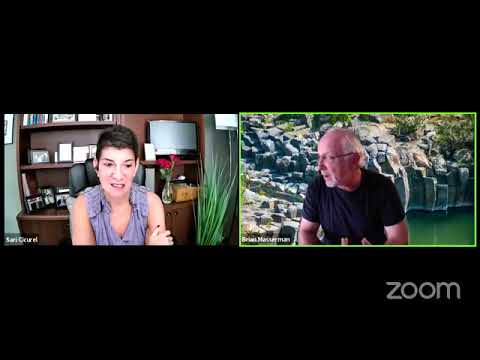This image is a screen capture of a Zoom conversation between two people, with black bars framing the top and bottom. The screen is split into two video images, featuring the participants.

On the left is a woman with short dark hair, wearing a purple, potentially sleeveless blouse. Her arms are crossed, and she is looking off to her left, focusing downward. Behind her is an office-like space with a wooden cabinet that has various items on its shelves, including a small video screen, a vase with red flowers, and a brown box. To her left, there's a green plant with long, wispy stems.

On the right side of the image is an older man with balding, white hair over his ears, white chin hair, and glasses. He's in profile, gazing to his right, seemingly at the woman. He wears a black t-shirt, and his chosen Zoom background depicts a natural pool area with dark green water and a rocky outcropping. The bottom portion of the screen includes the Zoom logo in the lower right corner.